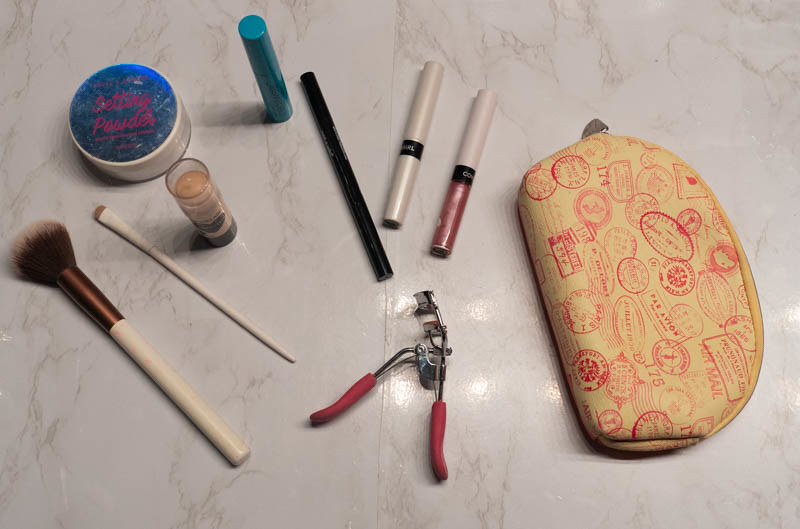In this detailed photograph of cosmetic accessories meticulously arranged on a countertop, the setting is a laminate surface with an off-white background subtly adorned with a marbleized pattern featuring light gray veins, touches of beige, and hints of mottled gold. The countertop elegantly reflects the light from six bulbs above, creating a soft, glowing ambiance.

To the far right, a distinctive yellow oval-shaped cosmetic bag catches the eye. It is adorned with various postage stamp-like seals printed in red, adding a whimsical touch. This bag zippers on the right, hinting at convenience and functionality.

Adjacent to the cosmetic bag are two lip glosses of the same brand, standing out with their distinctive packaging. These two glosses lie side by side; one displays a dark rose color contrasted by a white uppercase, with the rose shade filling in the lowercase. The other gloss comes in a completely white casing. Both feature black bands bearing a brand name that's not fully legible.

Next in line is an unsharpened black eyeliner pencil, its actual color veiled in mystery. Beside it, a sleek blue mascara, ready for use, stands upright. Flanking the mascara is a clear-cased concealer, also positioned upright, with its lower black end providing a striking contrast.

Above and adjacent to the blue mascara, a canister of setting powder is positioned. This white canister, crowned with a clear blue lid and adorned with pink lettering spelling “Setting Powder,” adds a vibrant touch. Below the setting powder, a makeup brush with a long white handle and camel-colored bristles rests elegantly, hinting at meticulous craftsmanship.

On the far left, another makeup brush designed primarily for powders makes its presence known. It features a white handle with a bronze-colored neck leading to a wide, soft brush head made from animal hair, promising a luxurious application experience.

Centrally placed in the lower third of the composition is a metallic eyelash curler with red handles, grounding the assortment of cosmetics with a touch of utility and style.